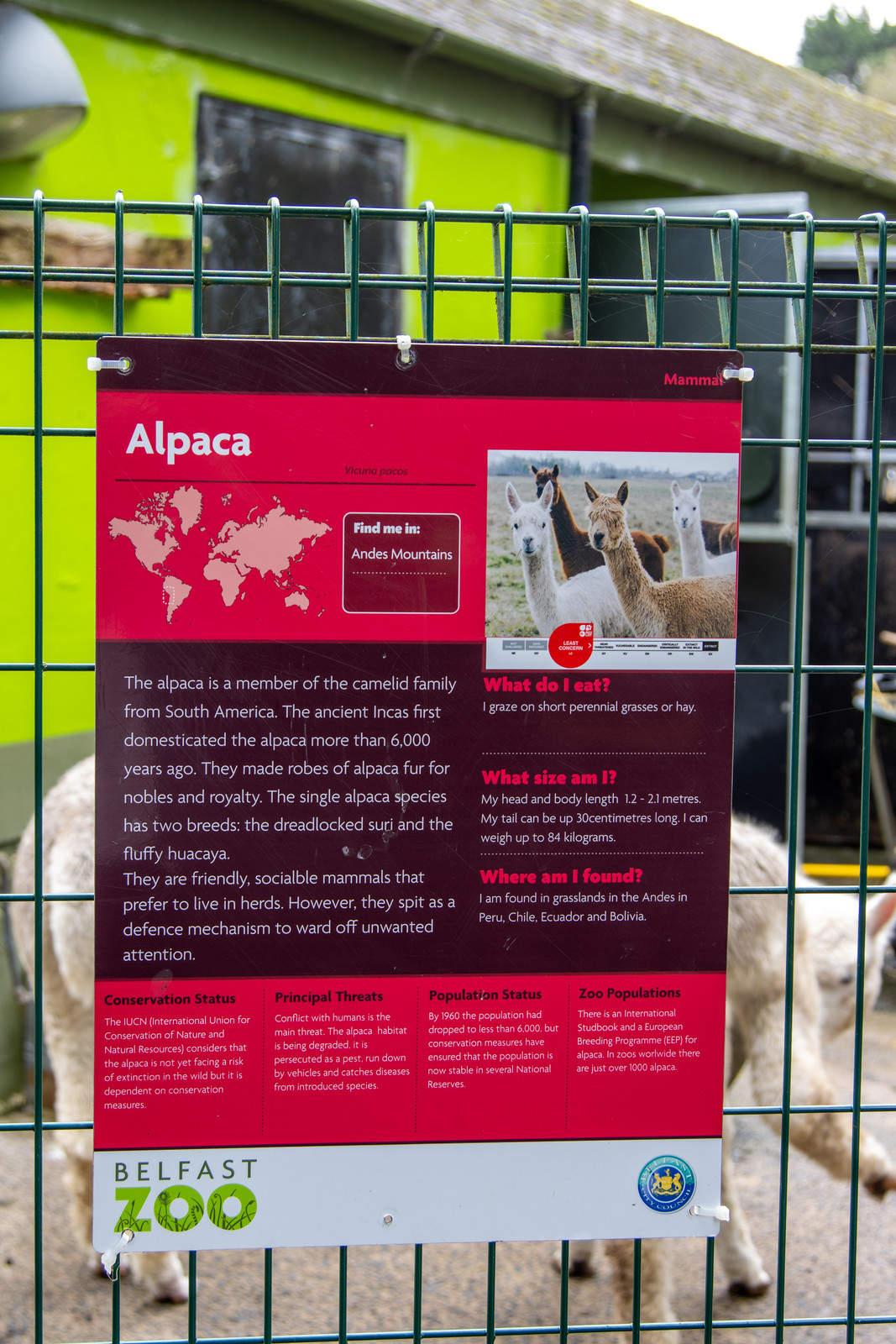The image features a red and deep red sign attached to the outside of a cage at Belfast Zoo. The sign prominently displays the word "alpaca" at the top in white text, accompanied by a partially highlighted world map indicating the native regions of alpacas, specifically the Andes Mountains. In the upper right corner of the sign, there is a picture of alpacas in the wild. Below this image, in smaller white text, there is a detailed description highlighting that alpacas are friendly and sociable mammals. The sign is divided into sections answering questions such as "What do I eat?", "What size am I?", and "Where am I found?". Additional information about alpacas' conservation status, principal threats, population status, and zoo populations is provided in the lower portion of the sign. The bottom left corner of the sign features the Belfast Zoo logo. Behind the sign, within the cage, faintly visible parts of a white alpaca can be seen—specifically, the legs and rear end—against a green backdrop that suggests the outdoor section of their display area.